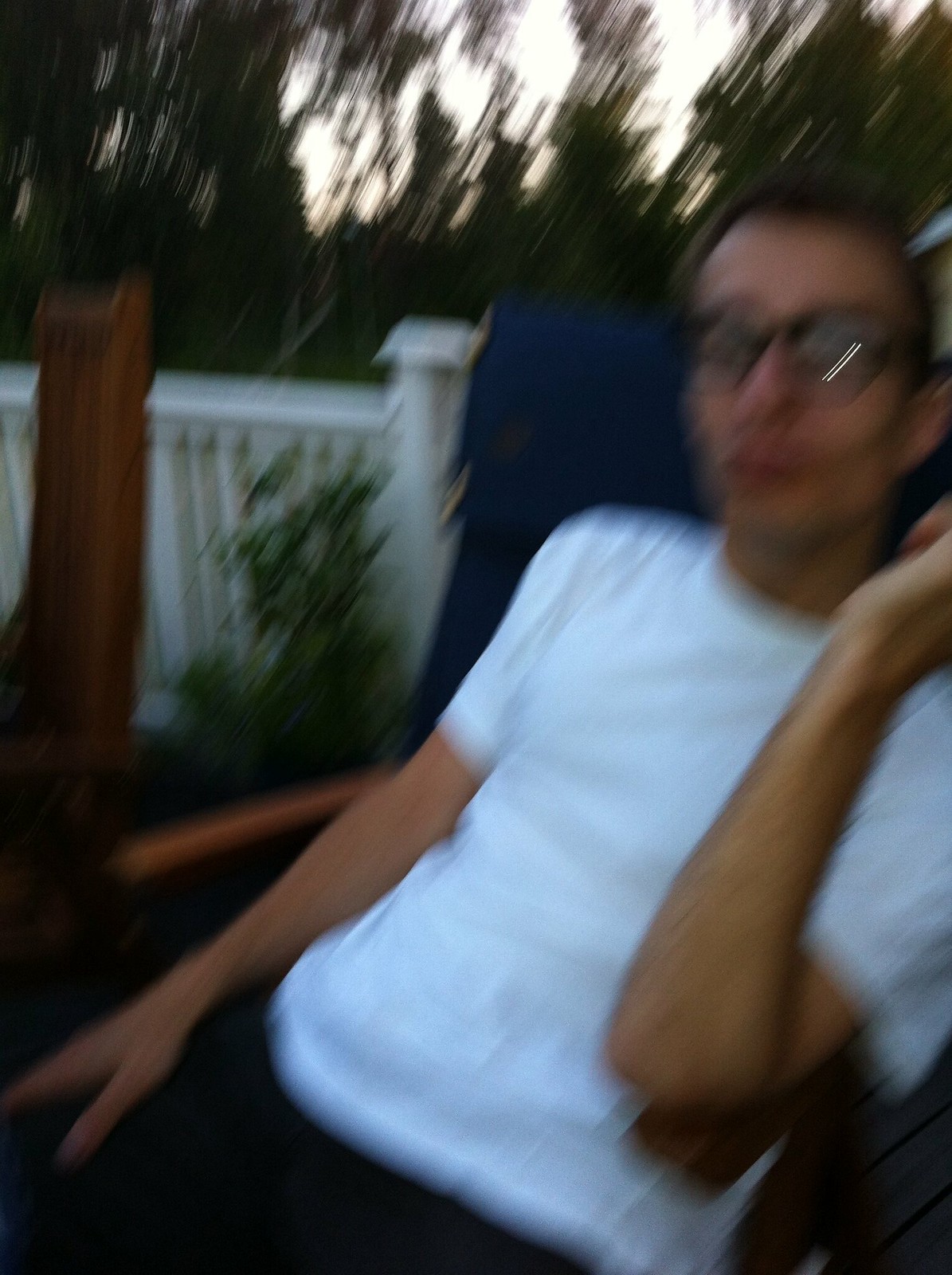In this blurry outdoor photograph, a male, possibly in his 20s or 30s, is seated in a chair and leaning back slightly. The subject is viewed from the front left, wearing a white t-shirt. Details of his pants are not visible, but his left hand is raised near his jaw, with the elbow at his side and fingertips out of the frame. He is wearing eyeglasses and has short, dark hair. His right hand rests on his right thigh. The background reveals various trees, patches of sky visible through the leaves, a white picket fence, and a large brown post of indeterminate purpose.